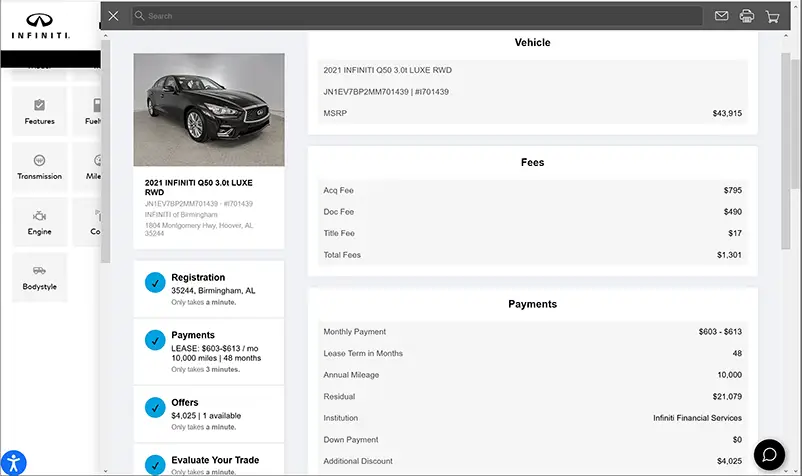This screenshot from the Infiniti website vividly captures a dual-layered user interface displaying key details and options for a particular vehicle. In the background, faintly visible, is what appears to be the main page of the Infiniti site or a detailed page for a specific car model. This page features a sleek white and black color scheme with various informational boxes outlining car specifications like features, transmission, engine, body style, and fuel information, though the overlay obscures some content.

In the forefront, the primary focus shifts to the detailed view of a specific vehicle: the 2021 Infiniti Q50 3.0T Luxe RWD. Prominently, a detailed list presents the car's Vehicle Identification Number (VIN), Manufacturer's Suggested Retail Price (MSRP) set at $43,915, along with additional pricing details including fees and payment options. 

On the top-left corner, a picture of the car showcases its design, immediately below which are the essential vehicle details. This leads into a checklist addressing various customer actions such as registration, making payments, available offers, and evaluating trade-ins. To enhance customer interaction, a speech bubble icon is positioned at the bottom right, suggesting an option to connect with a customer service representative for further assistance.

Overall, the screenshot efficiently combines aesthetic design with extensive information, creating a comprehensive and user-friendly browsing experience for potential Infiniti customers.